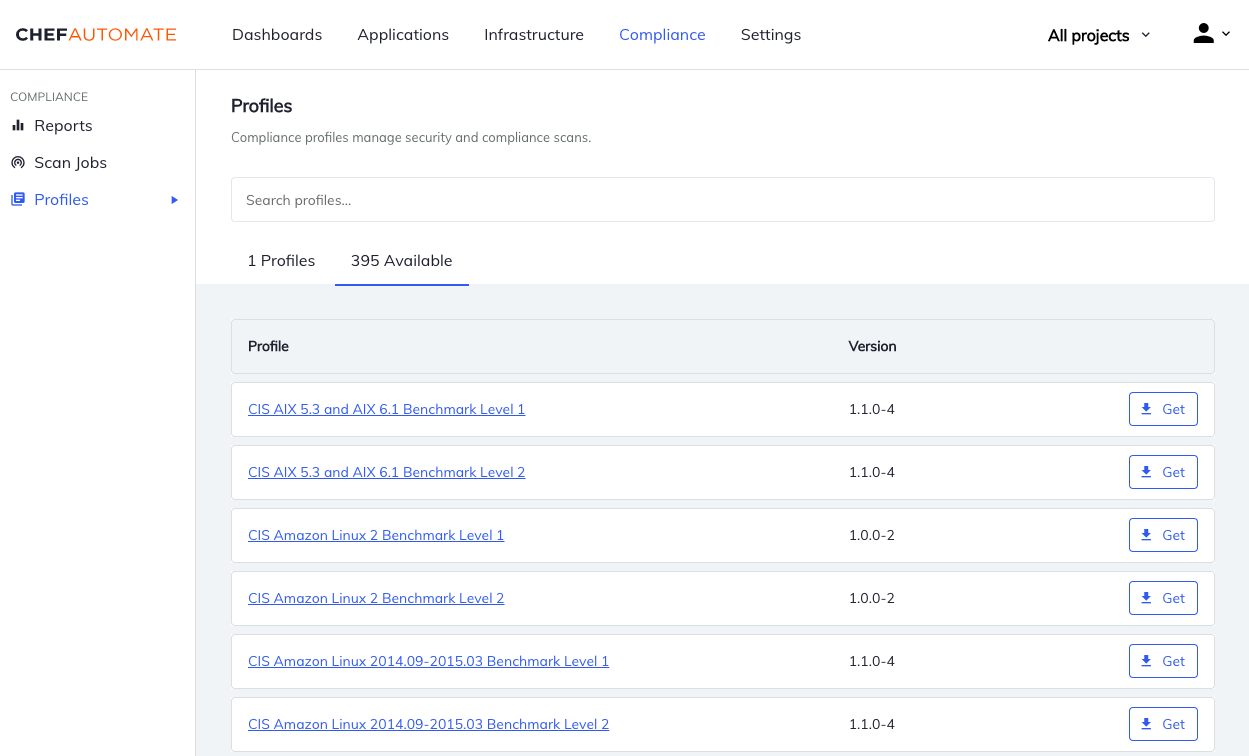Screenshot of the Chef Automate application interface, primarily displaying the Compliance Profiles section. The top navigation bar includes options for Dashboards, Applications, Infrastructure, Compliance (highlighted in blue), Settings, and All Projects, accompanied by a low-profile picture icon. The side menu lists Compliance, Reports, Scan Jobs, and Profiles, with Profiles highlighted in blue, indicating the current view. The main screen focuses on Compliance Profiles, which manage security and compliance scans, as suggested by an explanatory label. A search box is positioned at the top, revealing that 395 profiles are available. Visible profiles include titles such as "Benchmark Level One" and "CIS Amazon Linux 2 Benchmark Level One," followed by "Benchmark Level Two" and "CIS Amazon Linux Benchmark Level Two." The profiles contain symbols, letters, and numbers, hinting at intricate configurations pertinent to the Chef Automate application.